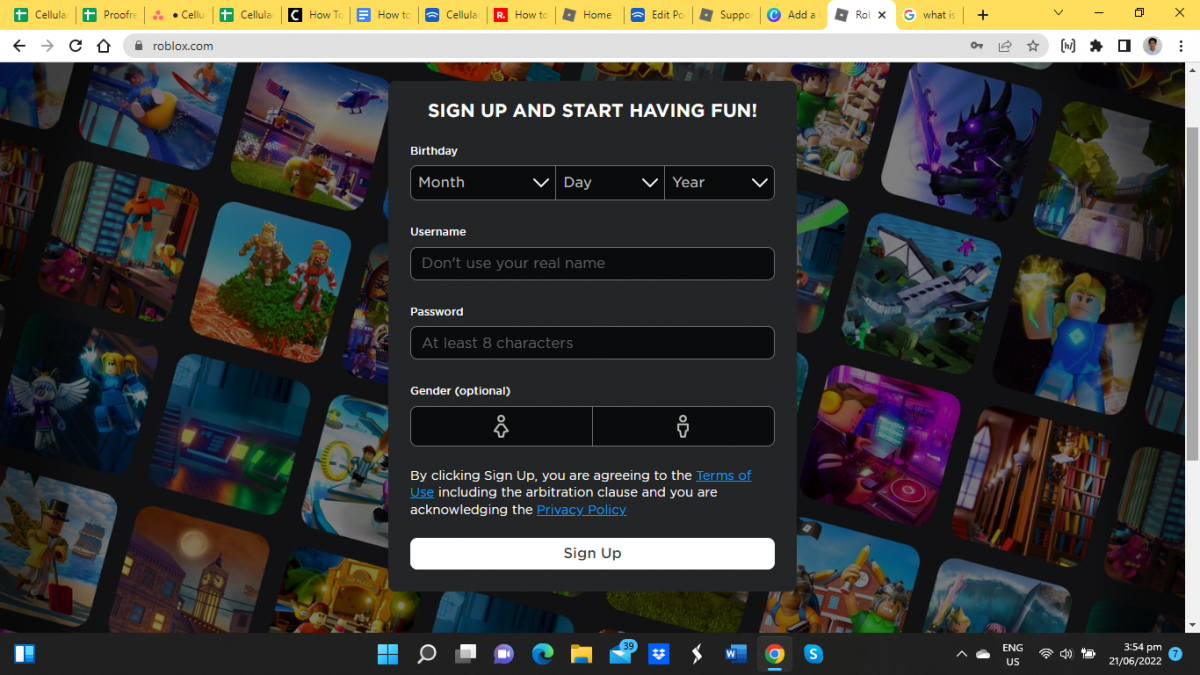This image is a screenshot taken from a web page open on someone's computer. At the top, there is a horizontal yellow bar displaying various open apps or tabs, highlighting the active tab in white, which is 'roblox.com'. Directly below this, there's a gray address bar where the URL is typed.

As you scroll down the page, the background is filled with numerous square images, each with rounded edges, depicting various scenes and characters from the Roblox game or related video games. These images showcase a diverse array of characters engaged in different activities such as holding spheres, flying, and standing on top of trees. The visuals are vibrant, featuring a wide spectrum of colors including red, yellow, orange, and shiny blue, which give an impression of electronic elements or covers. Additionally, one image features a moon, enhancing the variety of the scenes.

Centrally positioned on the page is a prominent black rectangle containing a sign-up section. This section invites users to "Sign up and start having fun" and includes a sign-up button, making it easily accessible for new users to join the Roblox community.